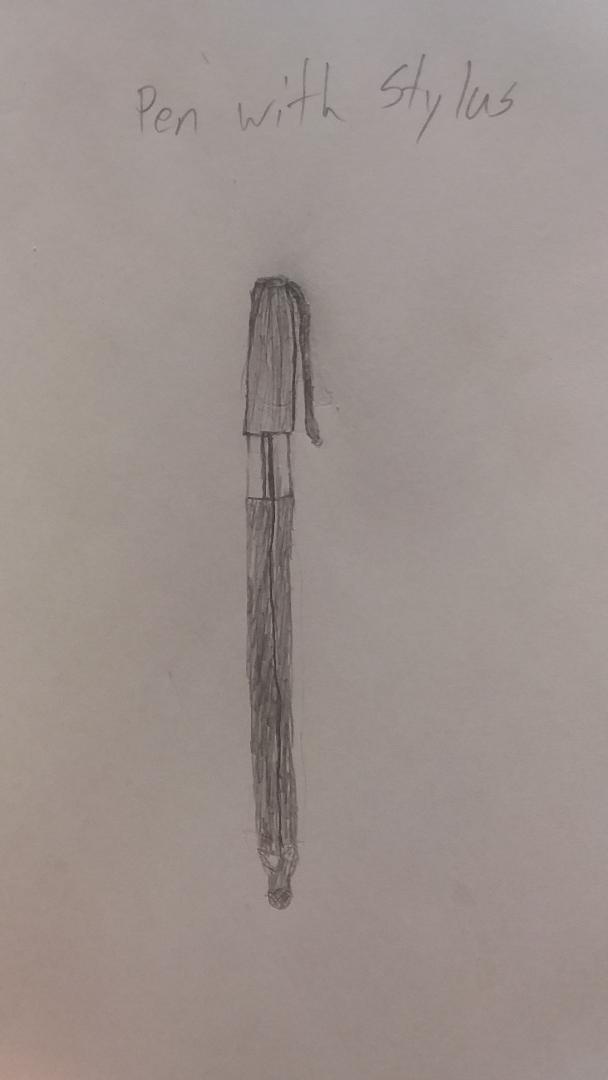A hand-drawn pencil sketch on a piece of white paper. The image is oriented vertically. At the top of the page, the words "Pen with Stylus" are written in an everyday pencil cursive. Below the heading, a drawing depicts a long, pen-like object with a pen cap at the top and a blunt, rounded bottom, indicating a stylus. The illustration is simple and not highly detailed, characterized by a uniform deep gray color with minimal shading, yet clearly identifiable as a hybrid pen-stylus.